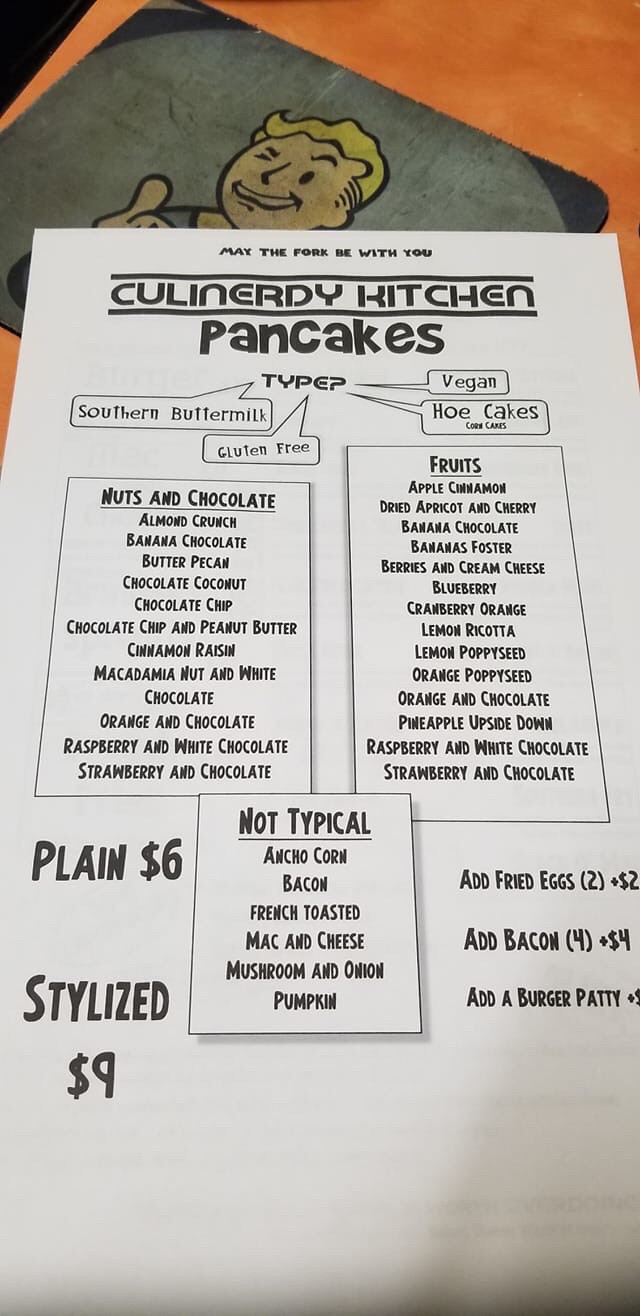The image is a color photograph presented vertically. At the top of the photograph, there is a salmon-colored surface, possibly a countertop or table. On this surface rests what appears to be a gray foamy mat, which could be an anti-fatigue mat. The mat has rounded, dark gray corners, and prominently features a black outline of a cartoon character with yellow hair, depicted winking.

Dominating the central area of the photo is a large white piece of paper, which appears to be a menu from Culinerdy Kitchen. The menu, titled "Culinerdy Kitchen Pancakes," lists various types of pancakes such as Southern Buttermilk, Gluten-Free, Vegan, and Hoe Cakes.

Below the type of pancakes, there is a section dedicated to different varieties featuring nuts and chocolate. Some of the options include Chocolate Chips, Butter Pecan, Almond Crunch, and Strawberry and Chocolate, adding up to about a dozen choices. This list is enclosed within a bordered text box.

Adjacent to the nuts and chocolate section lies another bordered text box listing fruit varieties available for pancakes. Options here include Apple Cinnamon, Strawberry and Chocolate, Lemon Poppy Seed, totaling around twelve varieties.

At the bottom of the paper, a small square bordered section is labeled "Not Typical." It lists unconventional pancake varieties such as Bacon, something Corn, French Toasted, Mac and Cheese, Mushroom and something, and Pumpkin. 

The bottom left corner of the menu indicates pricing: Plain pancakes are $6.00, while Stylized pancakes are $9.00. In the bottom right, there are options to add extras such as two fried eggs or bacon for an additional $4.00, or a burger patty for an undisclosed price.

The overall context suggests this is a menu from a restaurant specializing in diverse and creative pancake varieties, catering to a wide range of dietary preferences and tastes.